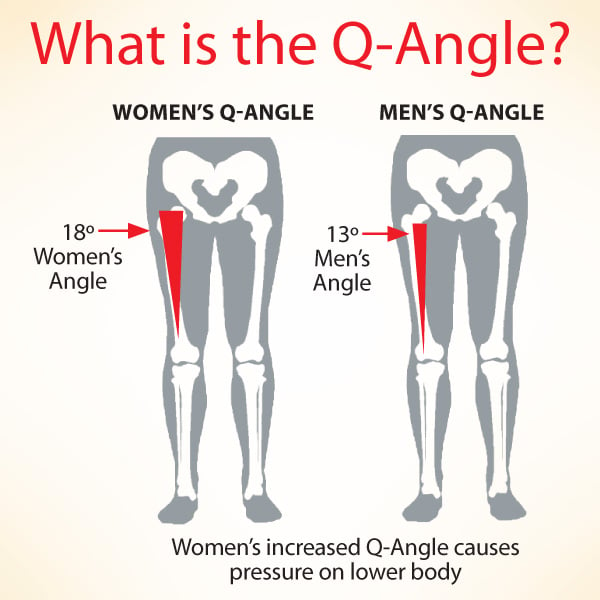The informational slideshow page is titled "What is the Q-Angle?" in large, centered red text. The background transitions from a light pink at the top to a mixed pink and white towards the middle and bottom. Below the title, the left side of the page features “WOMEN'S Q-ANGLE” in all caps, and the right side displays “MEN'S Q-ANGLE.” Underneath these headings, there are images depicting the legs and bones from the waist down for both men and women. According to the graphics, the women's Q-angle is indicated as 18 degrees with a red arrow highlighting the angle from hip to knee, while the men's Q-angle is shown as 13 degrees, also indicated by a red arrow pointing to the corresponding angle. The woman's Q-angle image is noticeably wider compared to the men’s. Centered beneath both pairs of legs, there is a caption stating, "Women's increased Q-angle causes pressure on lower body." The background varies slightly in description, appearing as an off-white or light tan shade.